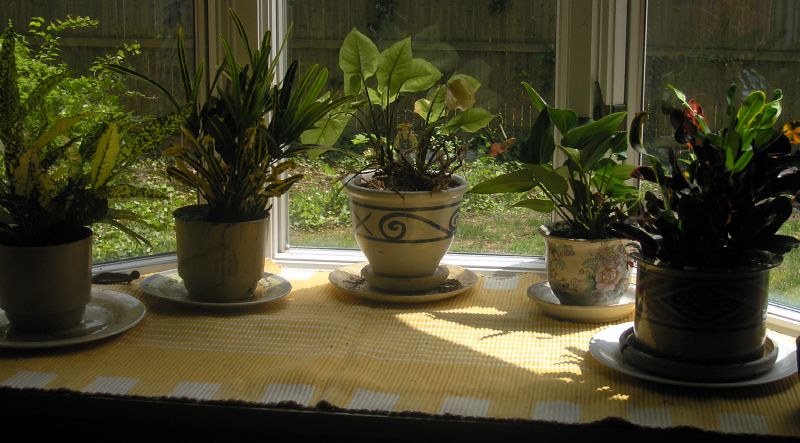The image captures a windowsill adorned with a yellow cloth featuring white squares, upon which sit five potted plants. The vibrant green foliage in each pot thriftily soaks up the sunlight streaming in from the top left, casting gentle shadows. From left to right, the first two plants are housed in plain brown pots with white saucers underneath. The central plant stands out in a white pot decorated with blue designs, while the fourth sits in a teacup-style pot with a painted flower motif, and the fifth, though dimly lit, shares a similar floral design. Through the window, there's a clear view of lush green grass and a wooden fence, suggesting a serene ground-level or basement setting.